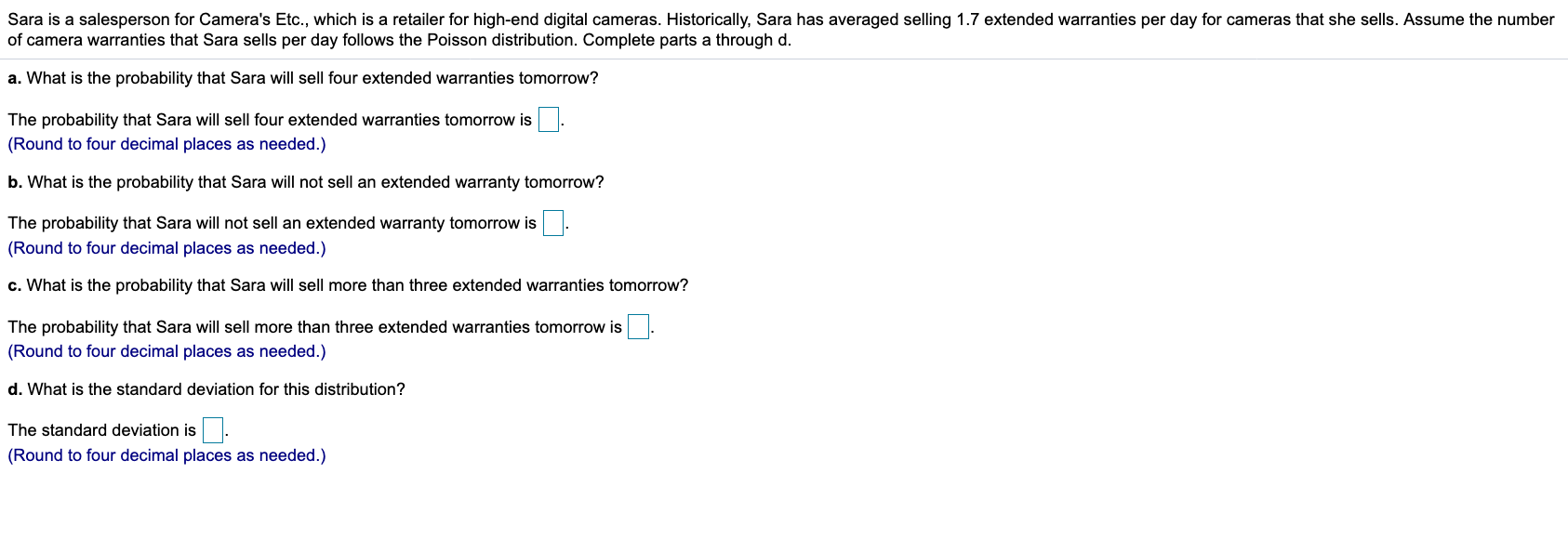**Detailed Caption:**

This image is a screenshot of a form designed to test statistical knowledge related to the Poisson distribution. The overall background of the form is white, and the text is predominantly in dark black font.

In the upper left-hand corner, the scenario is outlined: Sarah, a salesperson at "Cameras Etc."—a retailer specializing in high-end digital cameras—historically averages 1.7 extended warranties sold per day for the cameras she sells. The form assumes that the number of camera warranties Sarah sells per day follows a Poisson distribution. 

The form then directs the user to complete parts A through D:

- **Part A** asks: "What is the probability that Sarah will sell four extended warranties tomorrow?" A light blue box is provided for the answer, with instructions to "round to four decimal places as needed" in parentheses.
  
- **Part B** asks: "What is the probability that Sarah will not sell an extended warranty tomorrow?" Again, a light blue box is provided for the answer, with the same rounding instructions.
  
- **Part C** asks: "What is the probability that Sarah will sell more than three extended warranties tomorrow?" A light blue box is provided for the answer, accompanied by the same rounding instructions.
  
- **Part D** inquires about the standard deviation of this distribution, asking: "What is the standard deviation for this distribution?" A light blue box is provided for the response, with a note to "round to four decimal places as needed."

The blue boxes are meant for user input, ensuring responses are precise to four decimal places.